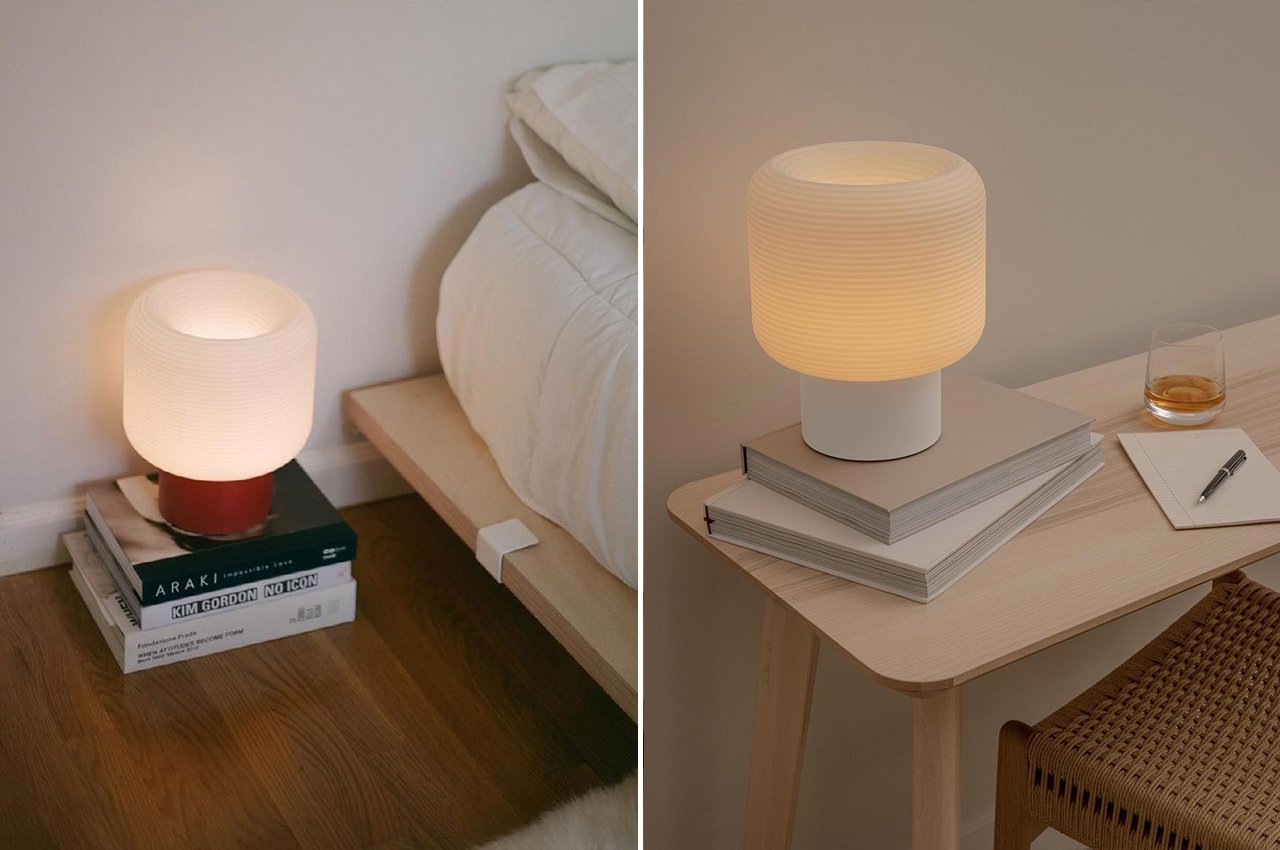The image features two similar-looking cylindrical lamps in separate settings. In the left picture, a large white lamp with an opening at the top sits on a stack of three textbooks on a wooden floor. The base of this lamp is red, and light is emanating from it. The background includes white walls and part of a bed with white sheets and a tan bed board partially visible.

In the right picture, a similar lamp with a white base and indentations of lines around it rests on two textbooks on a minimalist wooden desk. Nearby is a whiskey glass with an amber liquid, next to a yellow notepad with a pen on top. In the background, there is a brown wicker chair, and the wall appears to be a dark white to gray hue.